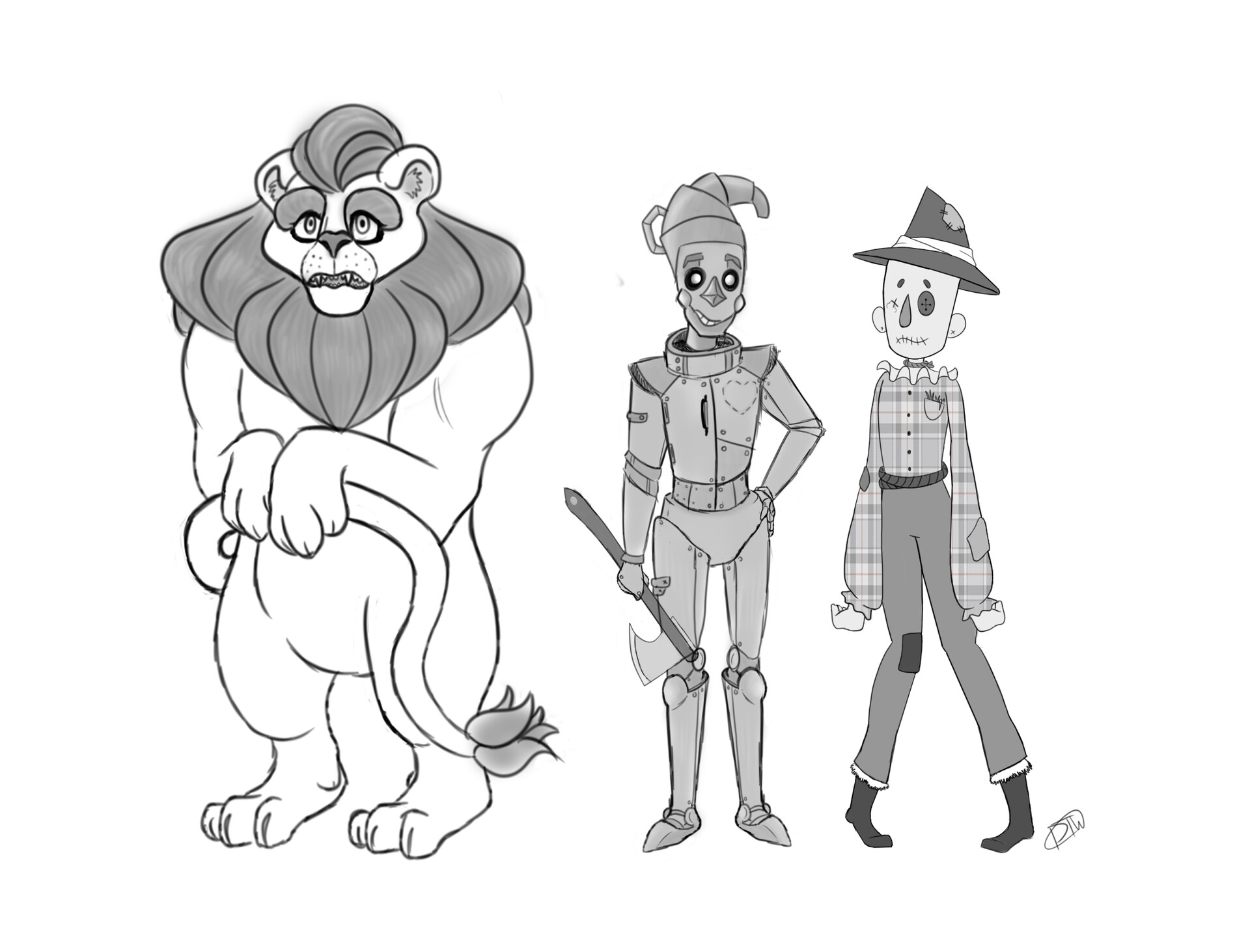This detailed monochromatic drawing depicts three stylized characters from the Wizard of Oz: the Cowardly Lion, the Tin Man, and the Scarecrow, each rendered with distinctive artistic features. On the left stands the Cowardly Lion, the largest of the trio, characterized by a white body, darker-shaded mane, and bushy tail he clutches in his paws, evoking an expression of shame or embarrassment. Positioned in the middle is the Tin Man, entirely shaded in gray, showcasing deep, sunken eyes and a comically exaggerated face. He brandishes an axe in his right hand, while his left hand rests on his hip, accentuating his armored appearance. Notably, a heart-shaped outline, marked by dashed lines, is drawn on the left side of his chest. On the right, the Scarecrow is portrayed wearing tattered, patchwork plaid clothing with an eye patch over one eye and an 'X' for the other, and his lips are stitched shut. He stands in a bowlegged posture, adding to his ragged appearance, with black socks and a white face completing his look. The overall composition offers a unique, stylized interpretation of these classic characters, with intricate details that distinguish each figure.